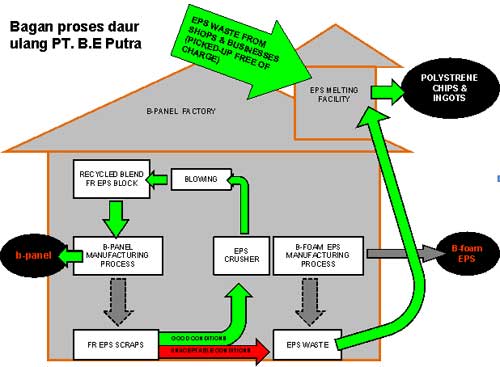The image is a detailed color illustration in a square format, depicting a flowchart of the waste management process inside a house, which is drawn in gray outline with an orange border. It features multiple arrows and labeled boxes describing various stages in the recycling and processing of EPS (expanded polystyrene) waste. At the bottom of the flowchart, a box labeled "FR EPS Scraps" is connected by a green arrow leading to an "EPS Crasher." From there, another green arrow leads upwards to a box marked "Blowing," which then guides to another side box labeled "Recycled Blend FR EPS Block." This box connects via a green arrow to a "B-Panel Manufacturing Process" box, which is then linked back to the first box.

At the top of the house, a prominent green box indicates "EPS waste from shops and businesses (picked up free of charge)," directing to a "EPS Melting Facility" labeled on a roof-like structure. Additional flowchart elements include a black ellipse on the right labeled "Polystyrene Chips and Ingots," showing a comprehensive flow of EPS waste from collection to recycling and repurposing. The illustration is captioned in a foreign language, providing a systematic view of the EPS waste cycle within a house-like structure. The overall style emphasizes a clean, organized flow of information with a clear progression from waste to recycled materials.